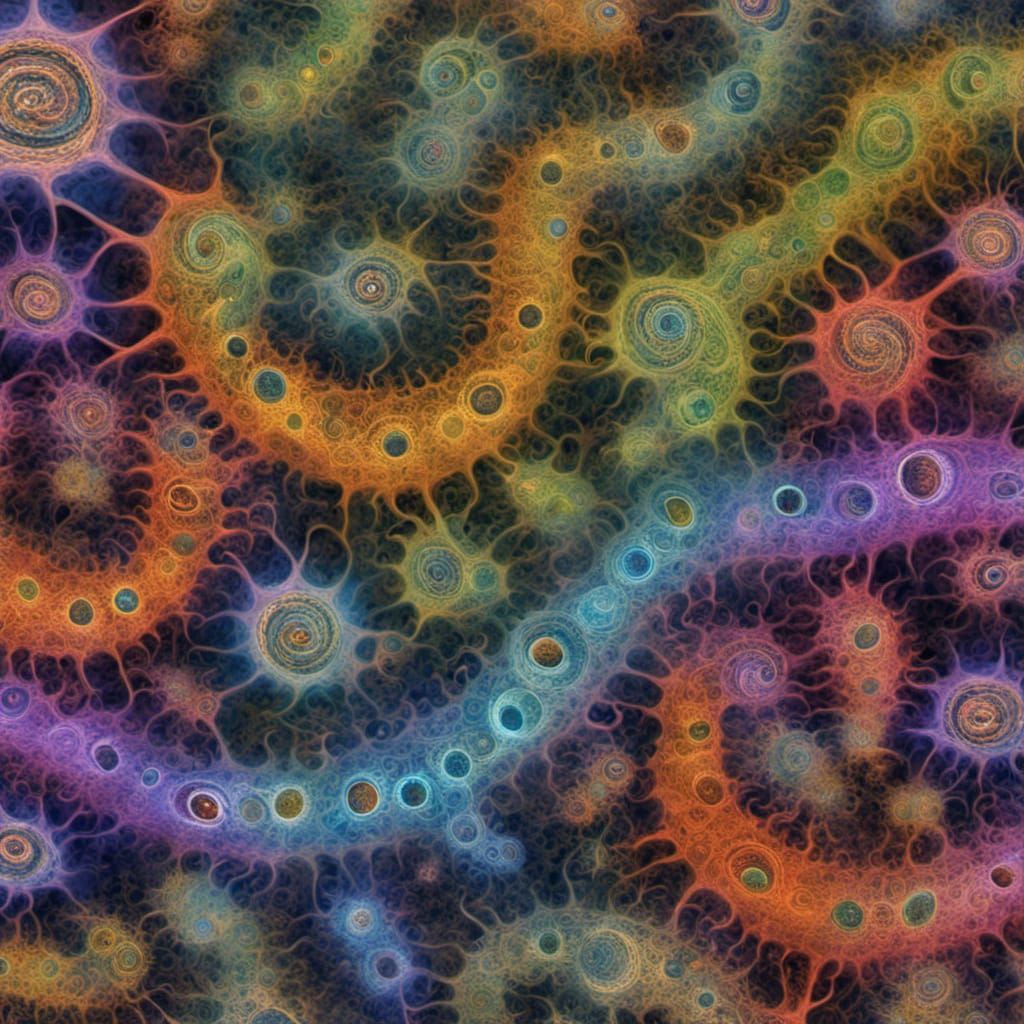The image is a highly colorful, intricate sketch that appears hand-drawn, set against a black background. It features a chaotic array of squiggly, worm-like shapes crisscrossing the page, accompanied by numerous small, circular forms. These shapes are vividly colored in hues of blue, red, yellow, orange, purple, green, and cyan. The worm-like figures and circles seem to interconnect with fine fibers, some resembling little ropes or snakes. The circles often contain swirly patterns and intricate designs, while the worm-like shapes may have holes with similar swirling interiors. The overall visual effect is reminiscent of a close-up rendering of bacteria under a microscope, with the black background speckled with fine fiber-like details adding depth to the complex, colorful scene.